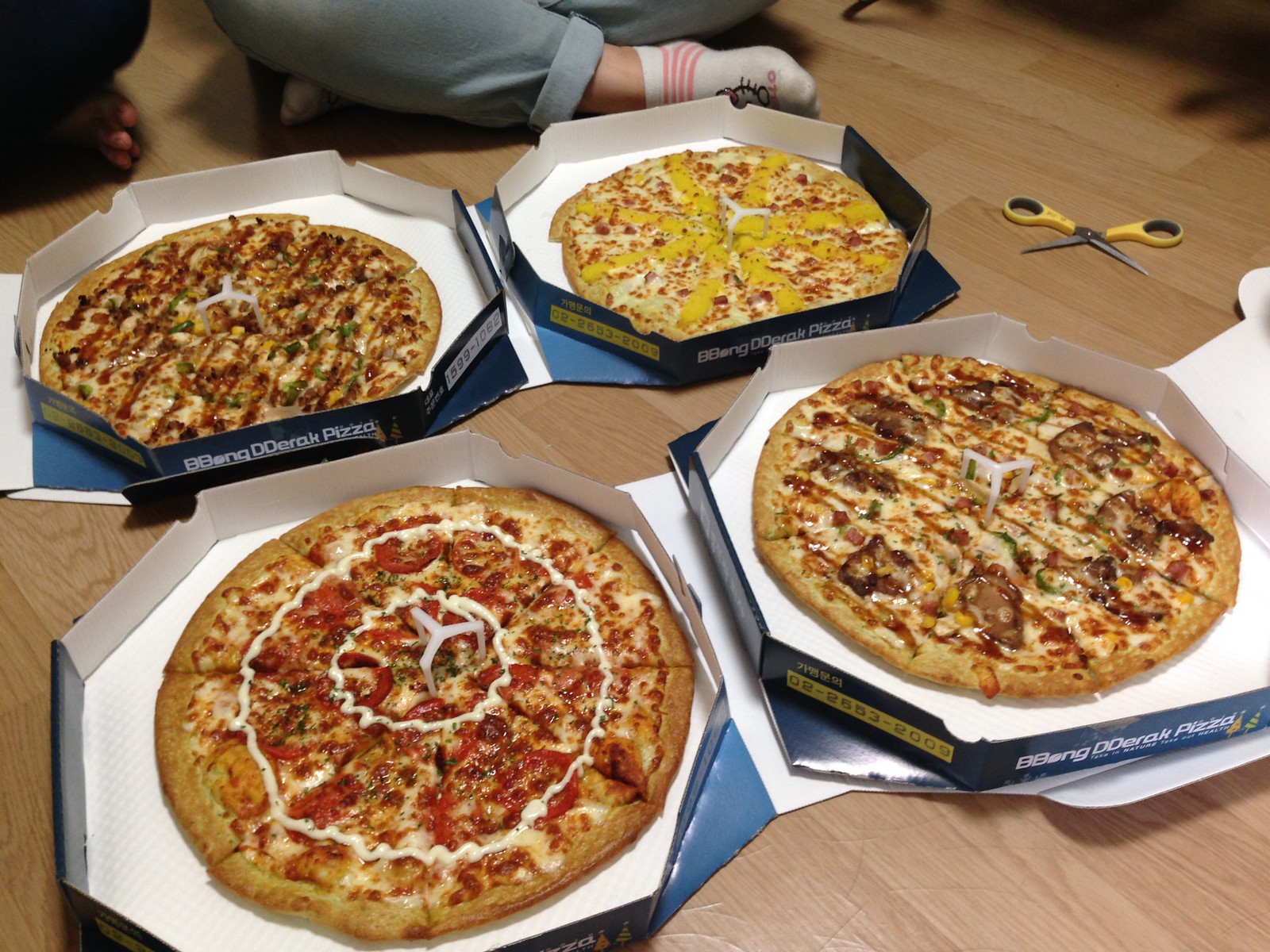In a detailed horizontal photograph, we see a wooden floor made of light hardwood panels, serving as the backdrop for a scene centered around four large pizzas in octagonal boxes. The boxes, open to display their contents, have a white interior and blue exterior, emblazoned with the white text "B-B-O-N-G-D-D-E-R-A-K pizza."

To the top left, two individuals are partially visible; one dressed in black pants with bare feet, and the other in gray pants and white socks. A pair of yellow-handled, stainless steel scissors lie open in the top right corner of the image.

At the center of the scene are the four pizzas, each with distinct toppings. One pizza appears to be a classic cheese variety with drizzles of white sauce. Another, positioned diagonally, features rows of banana peppers atop a cheese base. The third pizza has a thick crust, possibly adorned with a thin line of sauce resembling mayonnaise, and is topped with a mix of fruits, vegetables, and meats, reminiscent of a specialty pizza. The fourth pizza, with a thinner crust, seems to cater to meat lovers, scattered with pieces of steak.

Overall, the image artfully captures the pizzas in their boxes, the relaxed position of the individuals, and the scattered yet organized presence of the scissors, set against the light wood finish of the floor.